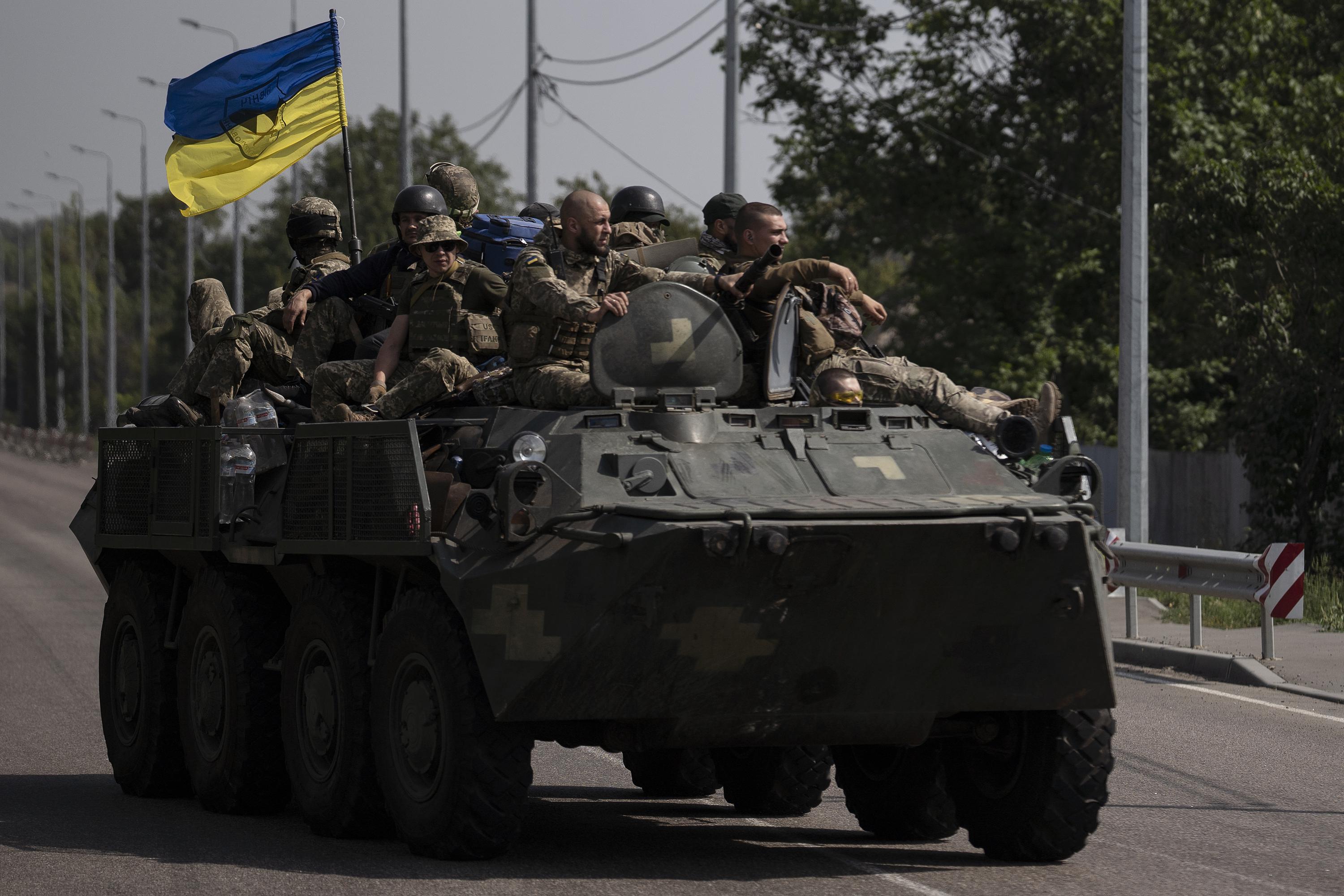The image depicts a large, greyish-black tank with eight wheels, moving down a deserted highway. The tank, which appears to be from a conflict zone, has the Ukrainian flag attached to the back. The flag, with its blue top half and yellow bottom half, features a prominent drawing of a face with black eyes. A total of ten soldiers, adorned in camouflage attire, are positioned on and around the tank. Some wear helmets, while others have hats. One soldier is visible through an opening in the tank, and another is seen holding what appears to be a gun. The environment includes power lines and tall street lamps lining the road, with scattered trees and an overcast sky in the background.